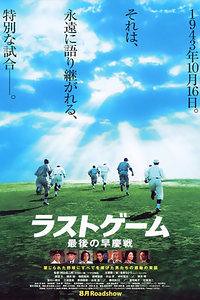The image depicts a vertical Japanese movie poster, adorned with vibrant details. At the top, a bright blue sky with scattered white clouds serves as a backdrop for four columns of vertical Japanese text. In the upper right corner, the year "1943" is prominently displayed. Below this sky scene, approximately seven individuals clad in white or grey uniforms, reminiscent of baseball gear or possibly prison attire, are shown running away from the camera across a lush, green grassy hill. Their shadows stretch beneath them, hinting at the sunny weather of what appears to be a summer day. At the bottom of the poster, the film's title and a byline are presented in Japanese, accompanied by photographs of the main actors and actresses alongside their names in smaller text. The word "Roadshow" is also visible at the very bottom of the poster.